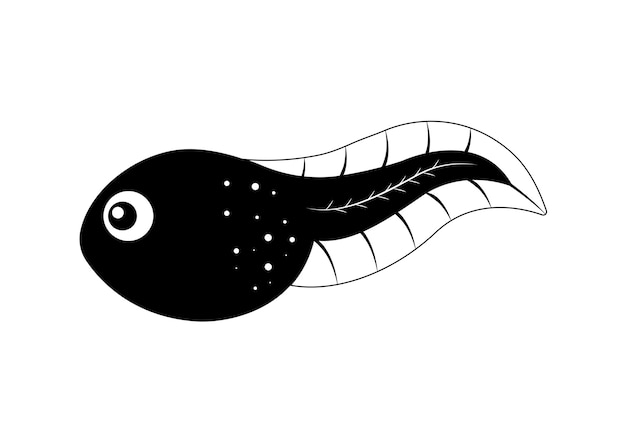The image is a simple, digitally created illustration in a black and white clip art style, depicting a tadpole. The tadpole faces left, appearing to swim in that direction, with a slight wave in its tail to suggest movement. It has a bulbous, oval-shaped black body transitioning into a long black tail of about the same size. The eye of the tadpole is striking, composed of a large white circle with a black pupil, which features a small white highlight dot. Just above the connection point between the body and the tail, there are several small white dots, possibly indicating shading. The tail itself has a central white line that resembles a fish bone, with smaller white lines branching off diagonally. Additionally, the tail is outlined by a thick white border featuring horizontal black lines, which gives the impression of a fin encasing the tail and adding to its overall size. The entire image is set against a plain white background, emphasizing the minimalistic and graphic nature of the artwork.